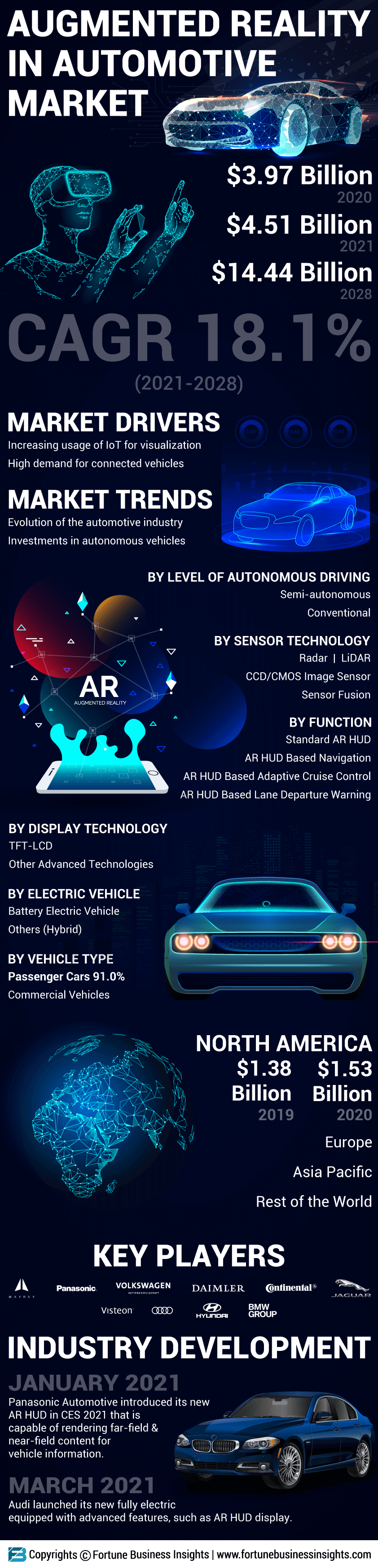The image is a long, dark blue advertising poster focusing on the augmented reality (AR) in the automotive market. At the top, in bold white letters, it reads "Augmented Reality in Automotive Market," accompanied by a bright line drawing of a futuristic car and an outline of a person wearing augmented reality glasses. The poster highlights several financial statistics: $3.97 billion in 2020, $4.51 billion in 2021, and a projected $14.44 billion in 2028, with a CAGR of 18.1% from 2021 to 2028. Key market drivers, such as the increasing usage of IoT for visualization and high demand for connected vehicles, and trends like the evolution of the automotive industry and investments in automotive vehicles, are outlined in white text. The poster also features images of cars, one in blue and another in smaller detail, and a blue line drawing of the Earth, specifically showing Africa and Europe. It highlights regional statistics for North America, with figures of $1.38 billion in 2019 and $1.53 billion in 2020. At the bottom, it mentions key players in the industry and notable industry developments from January and March 2021, though specific company names are indistinguishable.